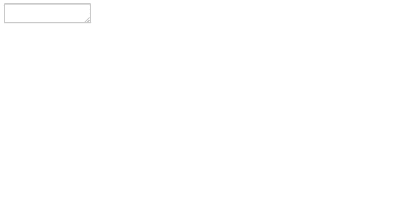The website appears to be non-existent, as the interface is largely empty. The background is predominantly white, creating a sparse and minimalistic appearance. In the top left corner, there are no messages or any written content. The main feature is a solitary message box situated in the middle of the page, and there is a pull tab located at the bottom right. Overall, the site offers very little information or functionality, with only the comment box and the pull tab standing out against the blank, unfocused white background.